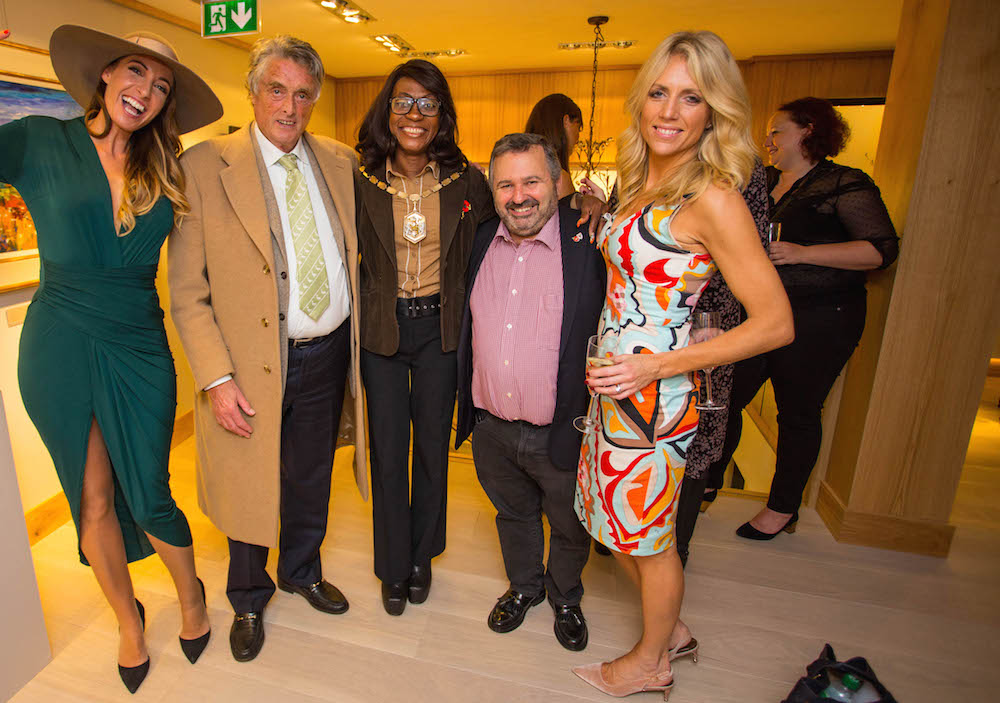This photograph captures a warm gathering of five individuals, likely taken in an office lobby or a boat's party setting, given the mix of wooden décor and a visible exit sign. From left to right, the group features a white woman in a green wrap-around dress with a high slit, plunging neckline, and a straw hat, smiling brightly. Next to her stands an older white gentleman with short, salt-and-pepper hair. He sports a camel-colored overcoat, a white shirt, a gray suit jacket, a golden tie, black pants, and black shoes. The third person is an African American woman with shoulder-length dark hair and eyeglasses, dressed in a brown jacket with a flower emblem, a tan shirt, black pants, and black clogs. Standing beside her is a short older man with graying hair, a mustache, and beard. He wears a pink shirt, a black suit jacket, gray pants, and black dress shoes. Completing the group is a younger white woman with dark-rooted blonde hair, clad in a vibrant, multi-colored dress featuring blue, red, orange, and yellow patterns, and holding a wine glass. The scene is lively, with two additional women in the background, one slightly heavier set in black pants and another with long black hair. The backdrop includes a yellow wall, wooden column, and a partially visible painting, highlighting the ambient and festive atmosphere.